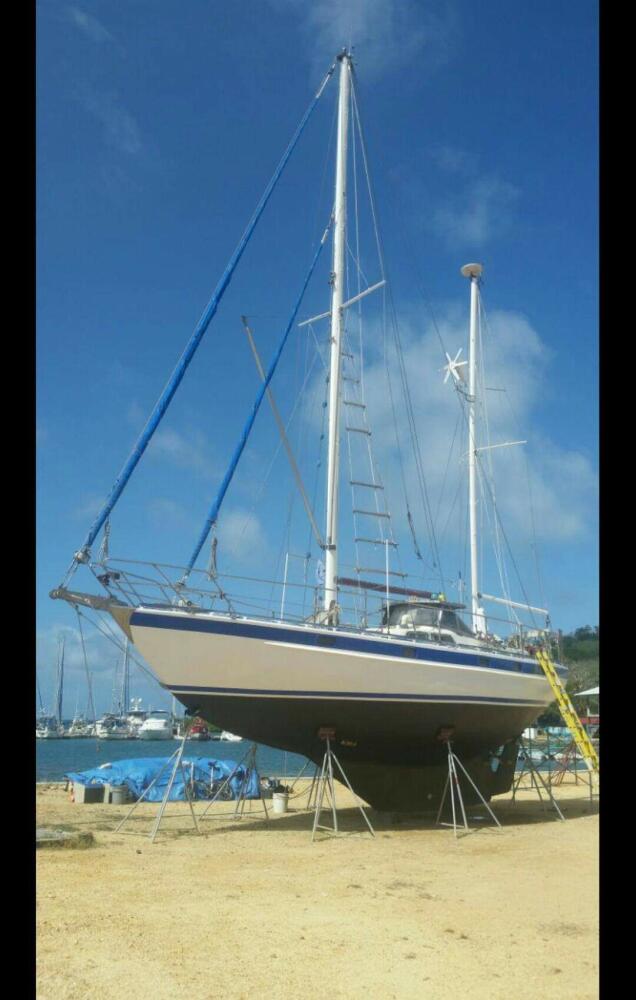The image depicts a large sailboat that is dry-docked on a beach or dockyard, supported upright by numerous light white metal tripod stands. The boat features a black hull transitioning to white sides with a thin blue stripe running along the rim. It has two tall white masts, anchored by various metal lines and blue ropes, one in the center and one towards the back, although no sails are set. A distinctive yellow ladder leans against the boat on the right side, providing access up the side, and a rope ladder is seen ascending one of the masts. The surrounding ground is composed of dry, loamy, yellow-brown dirt with no vegetation, suggesting a harsh, dry environment. The sun is high, casting a direct shadow beneath the boat, indicating it is midday. In the background, about 10 to 20 feet away, lies a harbor or marina with several other white sailboats moored in the water. The sky above is a crisp blue with wisps of thin white clouds, and a hill with some green grass is visible to the right. Notably, the image includes vertical black bars on either side, cropping the scene, and there are no people present.